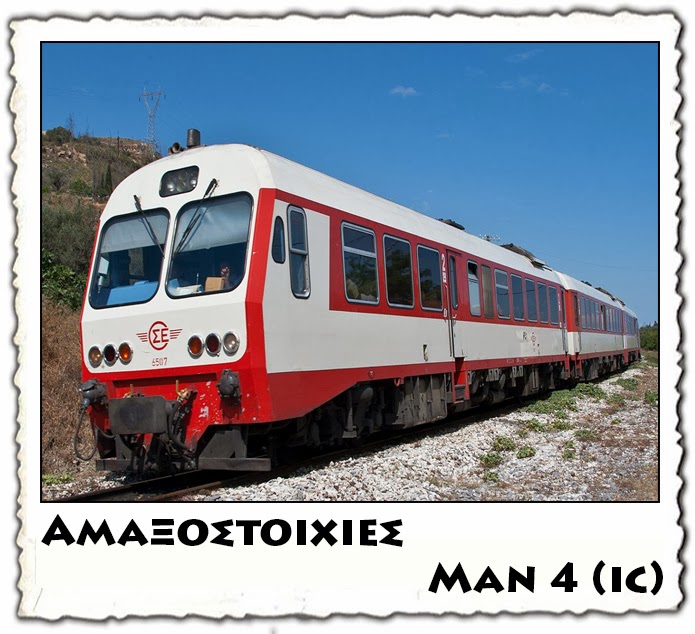The image depicts a white and red passenger train, three cars long, with the engine prominently positioned on the front left side and the rear of the train extending to the right-hand side of the photograph. The train is adorned with red trim along the bottom, front, and windows. A conductor's hand is visible through the right-hand window at the front. Above, the sky is a clear blue, and a large power line runs across the top of a hill in the left-hand background. The train is situated on tracks with white gravel pebbles nearby. Below the image, Greek text is written in block letters, while on the lower right side it reads "MAN4 (IC)" in English block letters.